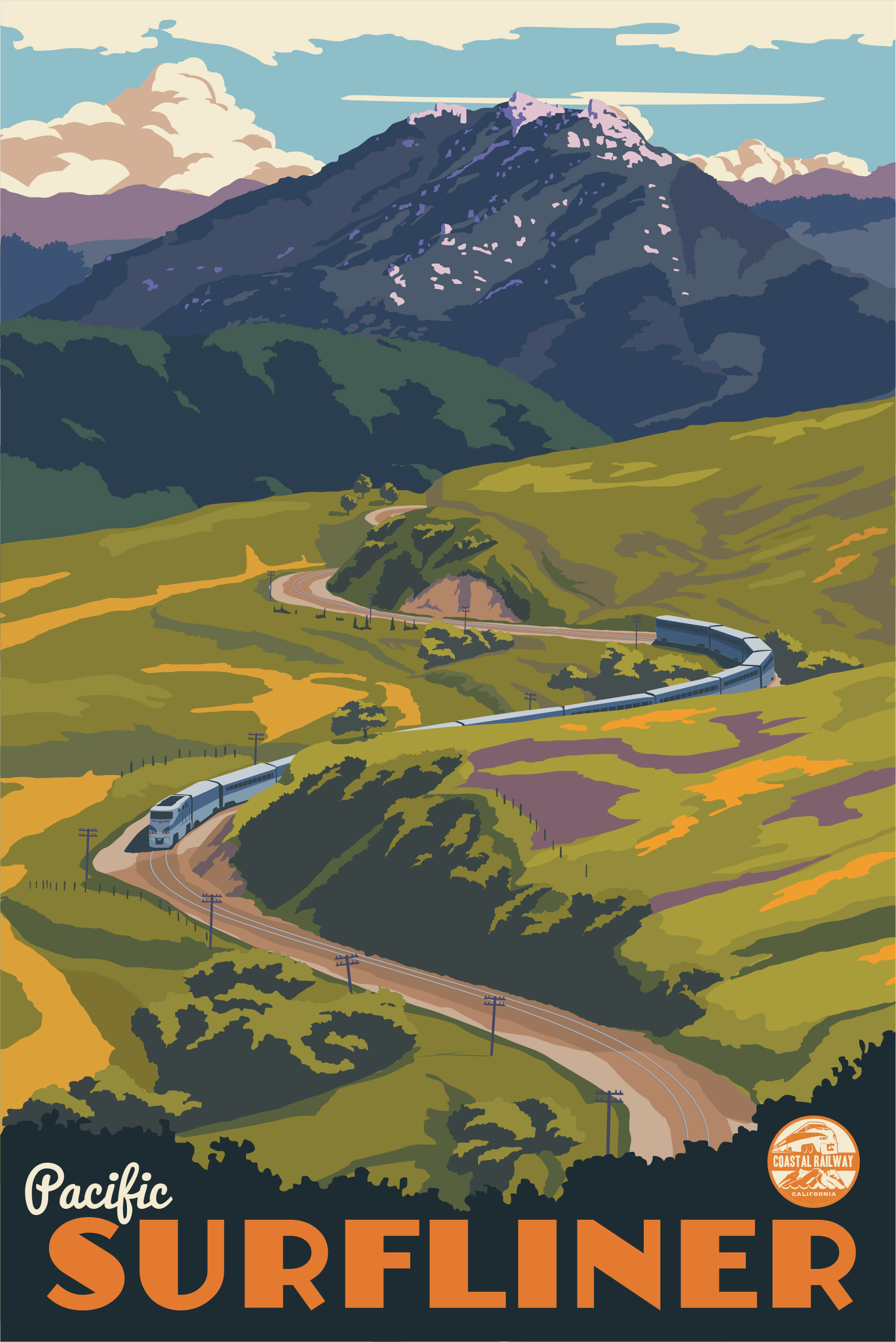The image is an artistic, vertically-oriented illustration resembling a postcard or poster. In the background, tall mountains, adorned with snow at their peaks, ascend into a sky dotted with clouds. A closer mountain, colored in shades of gray and rocky textures, stands before a lighter one, paired with grassy and potentially tree-covered hills. Descending these mountains is a curvy, winding S-shaped train track, leading towards the foreground and transitioning into a detailed depiction of a shiny, silver passenger train. This train, identified as the "Pacific Surf Liner," is highlighted by the text at the bottom of the image, with "Pacific" in white and "Surf Liner" in orange. The lower part of the image features a black silhouette of trees or bushes. Above all this, a circular stamp, possibly indicating "Coastal Railway" and hinting at a California location, is prominently displayed.